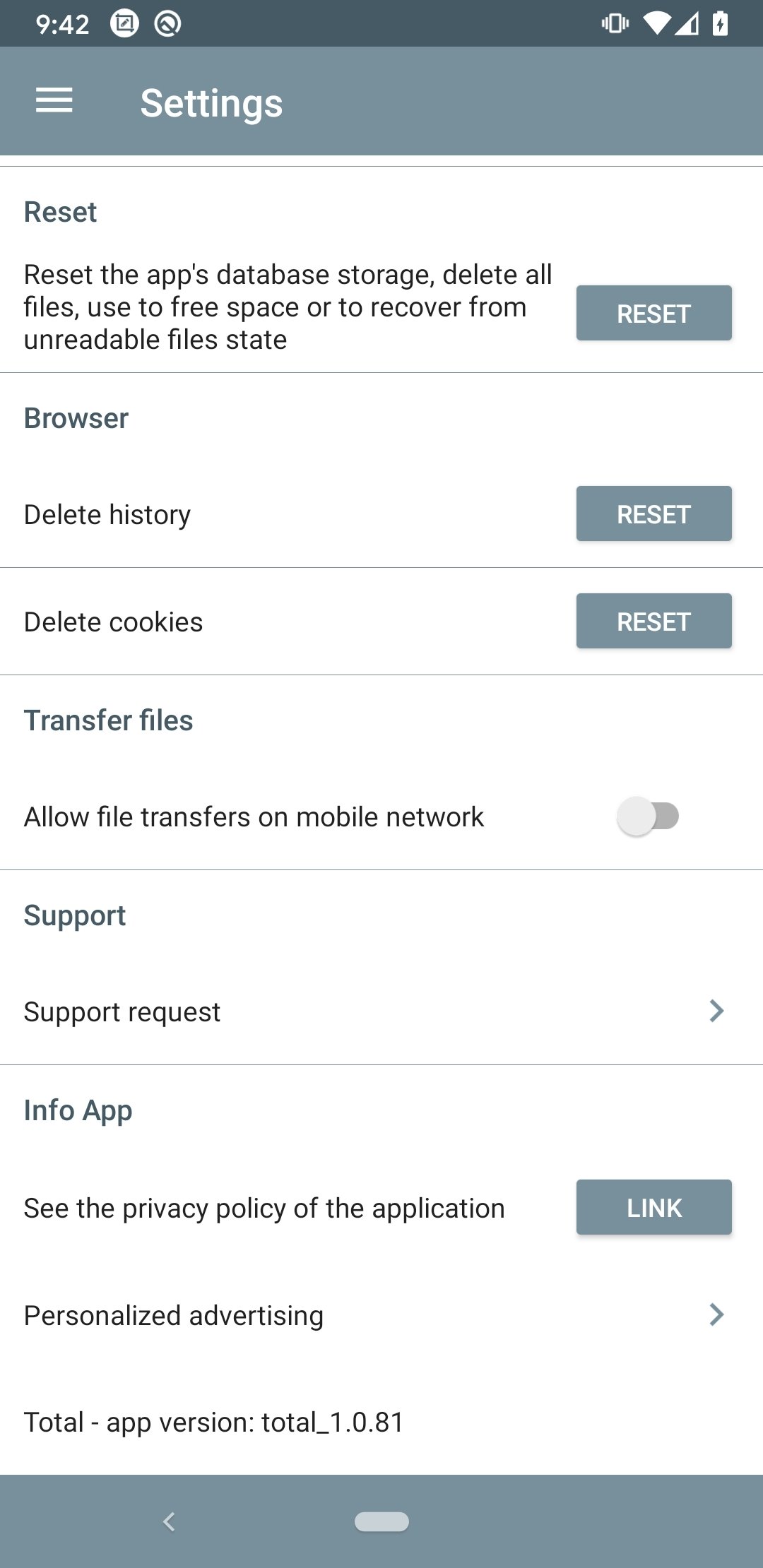Screenshot of a smartphone settings page.

The top border of the screen is dark gray, displaying the time as 9:42 (without indicating AM or PM) on the left side. The right side of the border shows icons for battery (with a charging indicator), Wi-Fi, and silent mode.

Below the top border, the header of the settings page is a medium to light bluish-gray color with the word "Settings" written in white on the left. To the left of this text are three horizontal white lines indicating the menu.

The main body of the settings page has a white background with organized categories:

1. **Reset**:
   - Description: "Reset the app's database, storage, delete all files used to free space or to recover from unreadable file state."
   - Action button on the right: A bluish-gray rectangle with the word "Reset" in white.

2. **Browser**:
   - Options: "Delete history", "Delete cookies"
   - Action button on the right: A bluish-gray rectangle with the word "Reset" in white.

3. **Transfer Files**:
   - Description: "Allow the file transfers on mobile network." (This option is set to "No" as indicated by the slider button being to the left).

4. **Support**:
   - Sub-option: "Support request" with an arrow pointing right, suggesting the presence of a dropdown menu.

5. **Info App**:
   - Description: "See the privacy policy of the application"
   - Action button on the right: A bluish-gray rectangle with the word "Linked" in white.

6. **Personalized Advertising**:
   - This section is simply labeled without additional detail.

At the bottom of the settings page, the footer shares the same bluish-gray color as the settings header. It also mentions the total app version as "total_1.0.81".